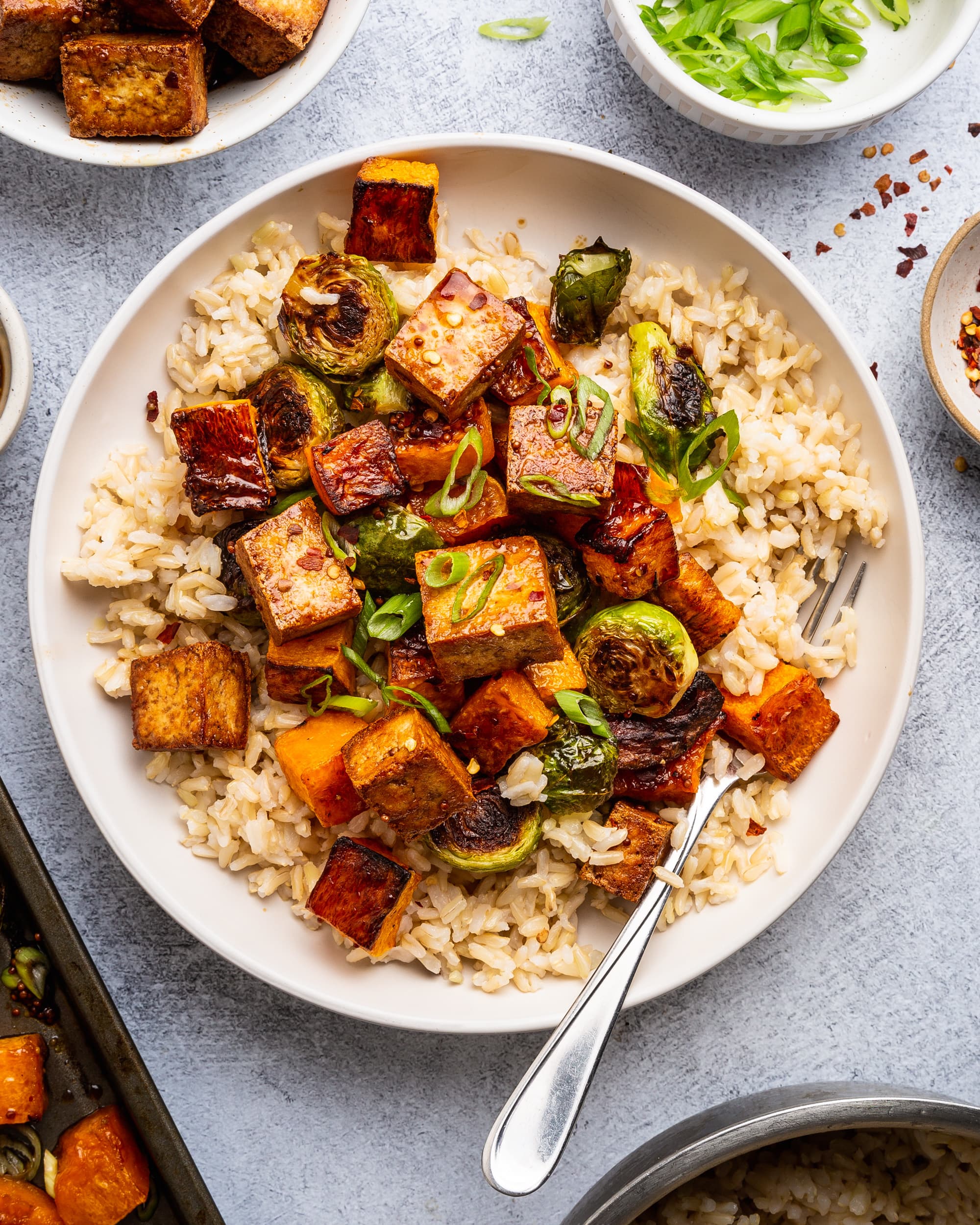This detailed top-down, color photograph showcases a beautifully arranged, healthy dish served on an ivory plate. The base of the dish consists of white rice, upon which sits an enticing mix of cubed sautéed tofu, roasted Brussels sprouts, and green onions. A silver fork is partially tucked under the rice and tofu, adding a touch of practicality to the plating. The dish is placed on a grayish table, surrounded by smaller, partially visible bowls containing additional ingredients like tofu, chopped green peppers, and rice, hinting at the meal's preparation and enhancing the overall composition.